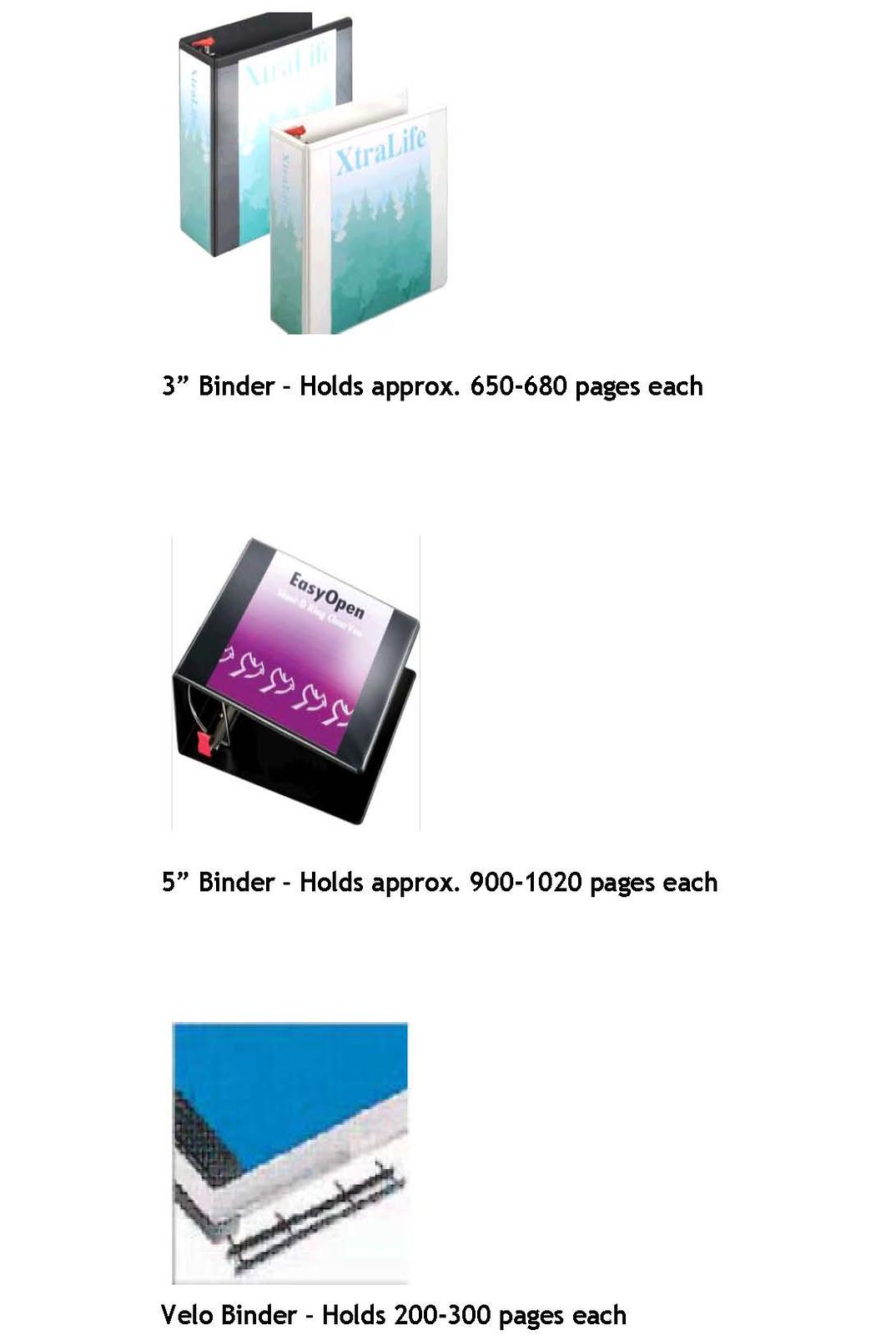This is a detailed image featuring three different types of binders against a white background. At the top, there are white binders with 3-inch spines, each capable of holding approximately 650 to 680 pages. These binders feature a light blue and green scenic design depicting a blue sky and evergreen trees, with the text "Extra Life" prominently displayed at the top. In the background, similar binders are shown in black, but with the same scenic image on them.

Below the 3-inch binders, a larger 5-inch black binder is shown, which can hold approximately 900 to 1020 pages. This binder features a purple label with the text "Easy Open." Some details on it are indistinct due to the image quality.

At the bottom, a Velo binder is displayed, which can hold 200 to 300 pages. This binder has a color scheme of blue with a black border, though the image is somewhat distorted, making it difficult to discern finer details.